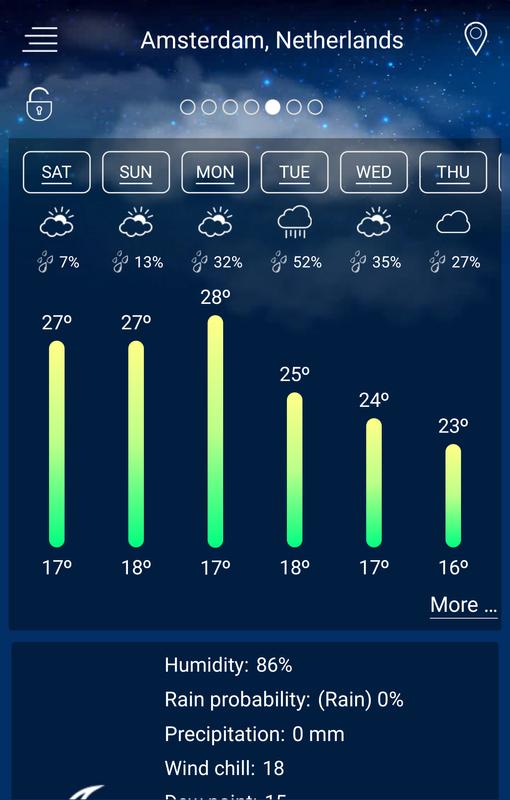**Weather Forecast for Amsterdam, Netherlands: Weekly Overview**

This screenshot from a weather app provides a detailed forecast for Amsterdam, Netherlands, displaying weather conditions from Saturday through Thursday. 

- **Location:** Amsterdam, Netherlands (Top right location pin icon)
- **Menu:** Additional options available (Top left with four lines icon)
- **Unlock Symbol:**
  
**Daily Forecast:**
- **Saturday:** Cloudy with a 7% chance of rain. Temperature ranges from 17°C to 27°C.
- **Sunday:** Partially sunny with a 13% chance of rain. Temperature ranges from 18°C to 27°C.
- **Monday:** Partially sunny with a 32% chance of rain. Temperature ranges from 17°C to 28°C.
- **Tuesday:** Rainy with a 52% chance of precipitation. Temperature ranges from 18°C to 25°C.
- **Wednesday:** Sunny with a 35% chance of rain. Temperature ranges from 17°C to 24°C.
- **Thursday:** Cloudy with a 27% chance of rain. Temperature ranges from 16°C to 23°C.

**Additional Information:**
- **Humidity:** 86%
- **Rain Probability:** 0% (for the current day)
- **Precipitation:** 0mm (for the current day)
- **Wind Chill:** 18°C